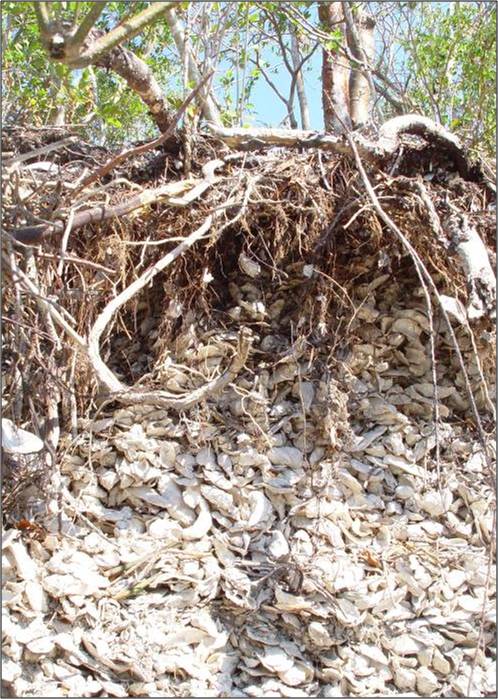In this outdoor image, the focus is on the intricate and exposed roots of a tree. The ground is slanting and scattered with numerous dead leaves and small rocks, which blend together under the diffused light. Amidst the chaotic tangle of the tree’s roots, dried twigs and vines intertwine, creating a complex mesh. The tree itself has a slim stem, and continuing up, you can see its branches extending outward. In the top left and right corners of the image, additional trees with lush green leaves are visible, providing a vivid contrast to the earthy tones below. The scene captures a rich tapestry of natural elements, from the ground up to the surrounding vegetation.